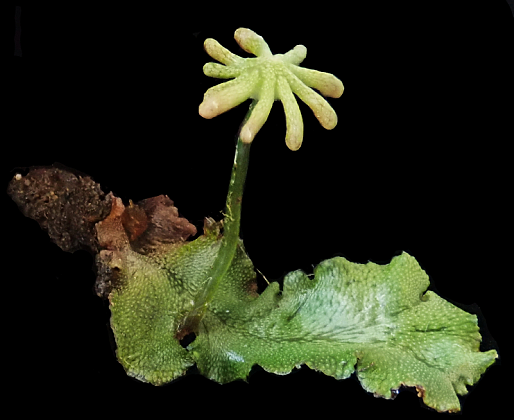This image showcases a meticulously detailed, intriguing structure set against a completely black background, creating stark contrast that emphasizes the subject’s peculiar appearance. Anchored in the upper left-hand portion of the frame, this feature starts with a base that appears brown, wilted, and decayed, suggesting organic degeneration or an artistic mimicry of such. Emerging from this base is a large, green, scaly leaf with a distinct white center and a rough, textured surface resembling the tongue of a cat. This leaf contributes an earthy grounding to the composition.

Rising from the center of this leaf is a green stem, noted for its somewhat transparent quality. This stem leads to the main attraction at the top – an unusual, flower-like structure. This 'flower' is a complex formation of yellowish-green tubular extensions, tinted with hints of pink at their tips. These extensions splinter outward almost like tentacles or the spindly ribs of an umbrella bereft of its fabric, imbuing the whole form with a whimsical, potentially otherworldly aura. The flower structure is light and almost ethereal in appearance, contrasting sharply with the more solid leaf base.

Permeating the entire image is a sense of ambiguity, leaving viewers to ponder whether they are observing a real botanical phenomenon or an abstract creation born from an artist's imagination. The organic, seaweed-like quality of the structure might suggest it could thrive in the mysterious depths of the ocean, adding to its enigmatic allure.